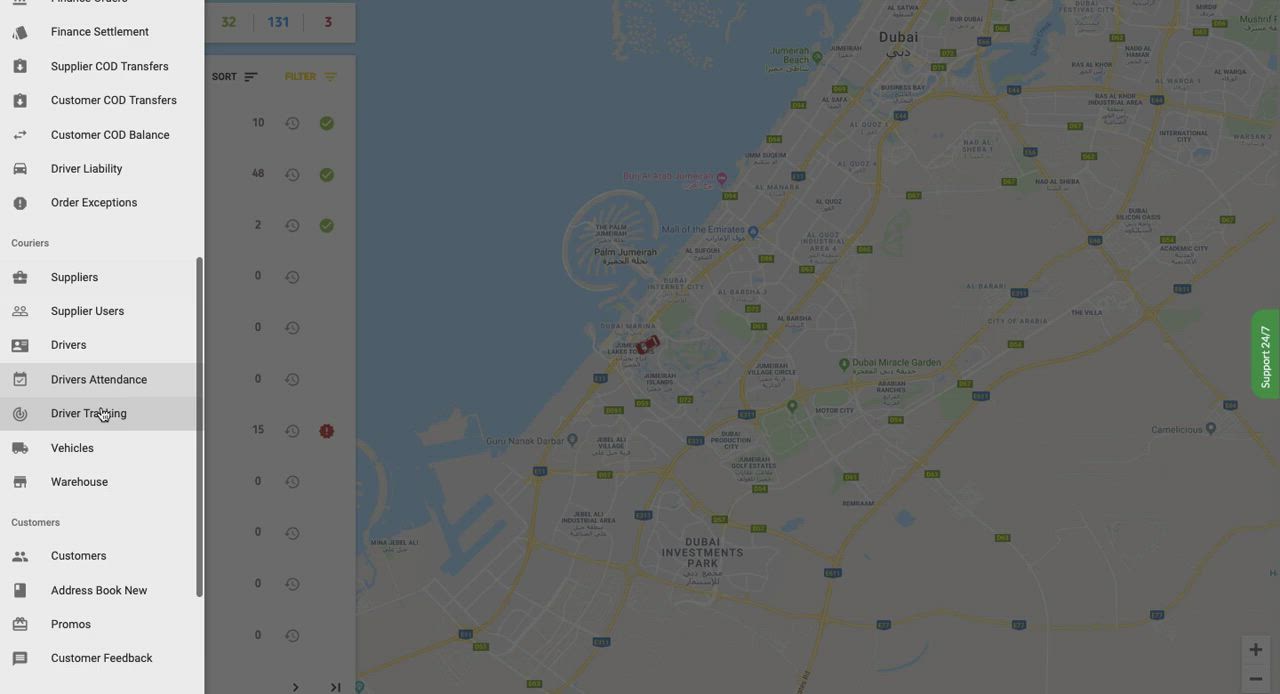The image is a screenshot of a GPS location application, resembling Google Maps, displaying an extensive menu bar on the left side. The menu bar, shaded in grey, contains a variety of options each accompanied by a relevant icon. The menu options listed are: Finance, Settlement, Supplier, COD, Transfers, Customer Transfers, Customer Balance, Driver Liability, Order Exceptions, Suppliers, Supplier Users, Drivers, Drivers Attendance, Driver Training, Vehicles, and Warehouse. For instance, the 'Vehicles' option has a truck icon next to it, and the 'Drivers' option features an icon of a driver's license.

On the right side of the screenshot, a large map of Dubai is visible, characterized by its distinctive tree island formation in the water. The map highlights different areas of the city, providing a detailed geographical overview.